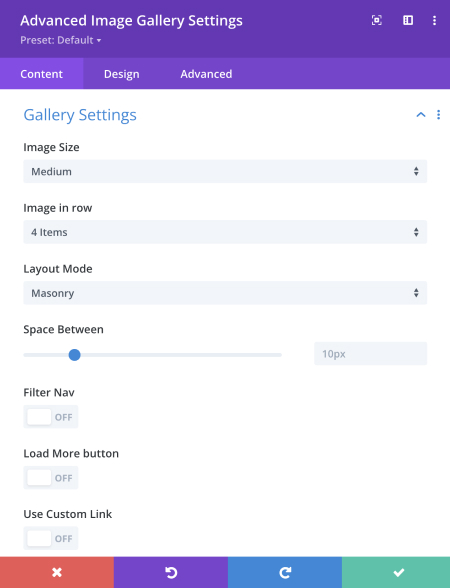Under the category "Websites," the interface displays a prominent purple bar at the top, labeled "Advanced Image Gallery Settings." This bar is followed by the text "Preset Default" and a dropdown menu for additional options. On the right side of this bar, three dots indicate a menu for more information.

Directly beneath this, there is a lighter purple bar with the labels "Content" (which is currently highlighted), "Design," and "Advanced," all written in white letters. The section following this bar is titled "Gallery Settings" in teal print, featuring a collapsible up arrow for navigation.

The "Gallery Settings" section details various options: "Image Size" set to Medium, "Images in Row" configured to 4, the parameter "Items" present without a specific value, "Layout Mode" set to Masonry, and "Space between" adjusted to 10px. Additionally, both the "Filter Nav" and "Load More Button" features are turned off.

At the bottom of this configuration panel, there are four distinct buttons: a red rectangle with a white X, a purple rectangle labeled "Go Back," a blue rectangle labeled "Go Forward," and a very light green rectangle containing a white checkmark.